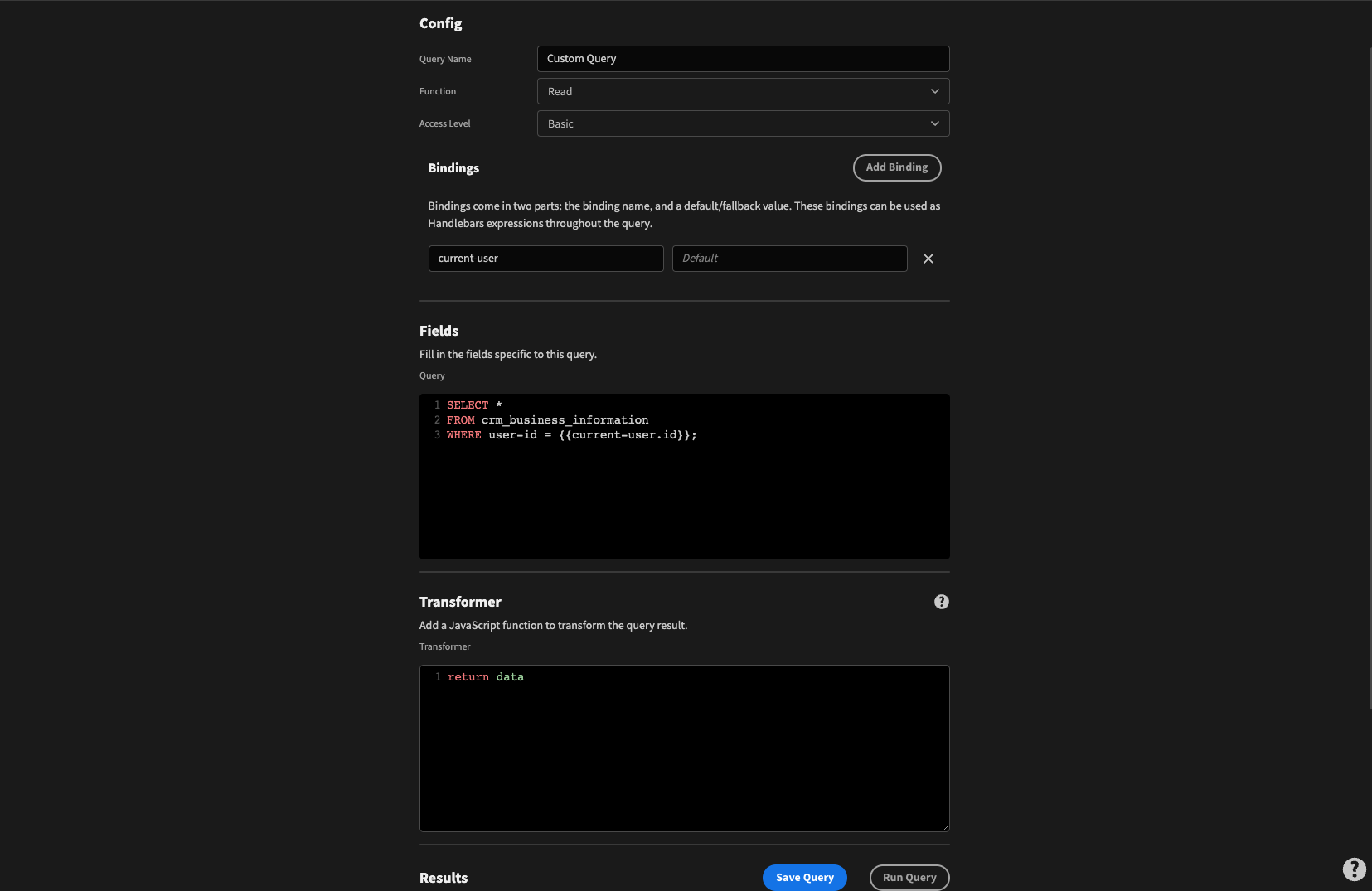The image features a predominantly black background with varying shades, creating a matte finish transition towards the edges. At the center, there are three distinct panels, each containing detailed configurations and options.

The topmost panel is titled "Config" and includes fields labeled "Query Name," "Function," and "Access Level," all of which have been populated with data. The "Query Name" field reads "Custom Query," while the "Function" and "Access Level" fields display "Red" and "Basic," respectively.

The second panel is labeled "Bindings" and offers an "Add Binding Option." Below this, a section is devoted to the "Current User," labeled as "Default." A horizontal line separates this section from the following fields. The section is titled "Fields" in white text, instructing users to "fill in the fields specific to this query," followed by placeholders "Select, From, Where."

The third panel, titled "Transformer," prompts users to "Add a JavaScript function to transform that query result." It displays a coding area with a black background featuring the text "Return Data." The term "Return" is highlighted in red, while "Data" appears in green.

At the bottom of the image, there is a section labeled "Results," displaying a blue tab named "Siri Query" followed by an option to "Run Query." In the lower left corner, another "Results" section is signaled.

This detailed configuration interface appears to be part of a software application designed for managing and executing custom queries and transformations.